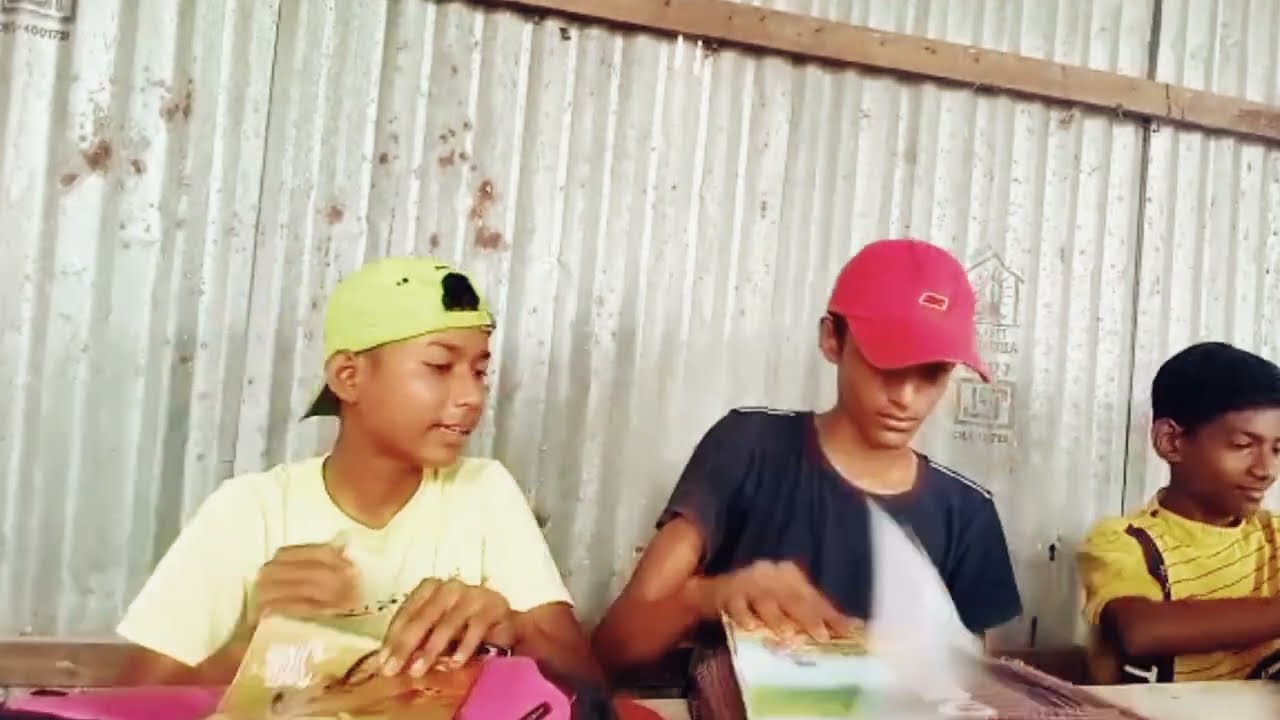The photo captures three young Indian boys, likely aged around 11 to 13 years old, sitting at a table in front of an old, weathered wall made of corrugated sheet metal with a tarnished, potentially copper cross beam. The boys are engrossed in various magazines or paper-based reading materials. The boy on the left, wearing a yellow shirt and a light green baseball cap turned backwards, is about to turn a page while glancing over at his friend's magazine. In the center, the boy with a dark blue shirt and a white baseball cap appears focused on his own magazine. The boy on the right, dressed in a black and yellow striped shirt, seems somewhat detached from the others' activities. Despite their varying levels of engagement, all three seem to be enjoying their time together in this rustic setting.